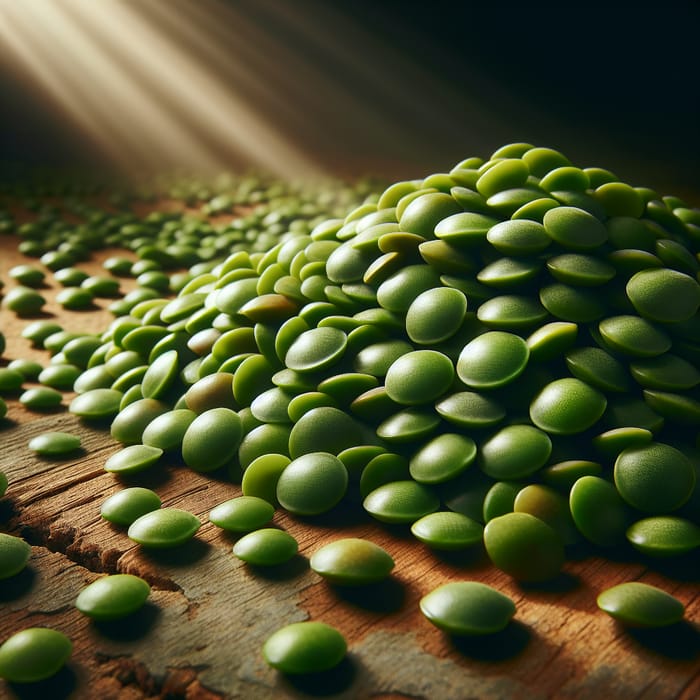The image showcases a vast array of small, bright green orbs that closely resemble lentils or peas but with an unusual, flat, flying saucer-like shape, suggesting they might be artificial or AI-generated. These orbs, numbering in the hundreds or thousands, are scattered loosely and stacked high on the right side of a rough-hewn, old, and cracked wooden tabletop in worn tan and rusty brown hues. Light beams from an unknown source outside the frame illuminate the scene, casting light on the table and causing subtle reflections on the green orbs. The background transitions from black to dark brown, fading into rust brown near the light beams in the top left corner. Some of the orbs exhibit yellowing, implying they might be aging or decaying. The overall appearance is a detailed, almost surreal depiction, with every minute detail of the orbs and the table surface vividly captured.